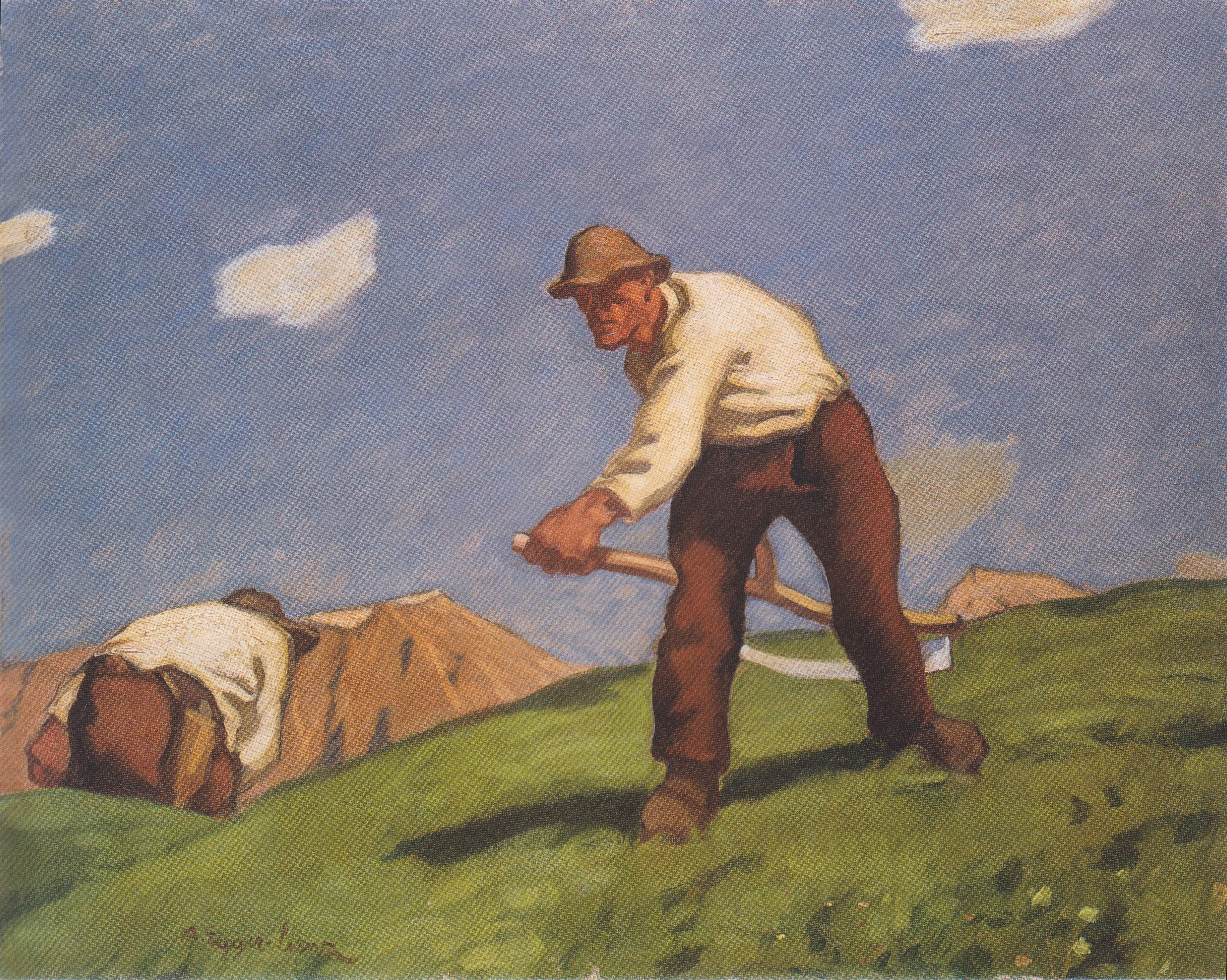This detailed painting, done in the Impressionist style, depicts two men laboring in a grassy hillside field, with a backdrop of mountainous terrain. The central figure, dressed in a white long-sleeved peasant shirt, brown pants, and brown boots, is portrayed bending over with a tan-handled sickle ready to cut the overgrown grass and weeds. He wears a lighter sandy-colored brown hat. Beside him, a second man, seen from behind in an identical outfit, also engages in the same laborious task. Their surroundings include a mix of green hills and another range of dirt-colored mountains adorned with some snow caps in the distance. The blue sky above is scattered with both white puffy clouds and a distinctive gray cloud hovering above a mountain peak to the right. Small flowers are interspersed within the grassy field, and a signature, though not legible, is located in the bottom left corner of the painting, adding a final touch of authenticity.